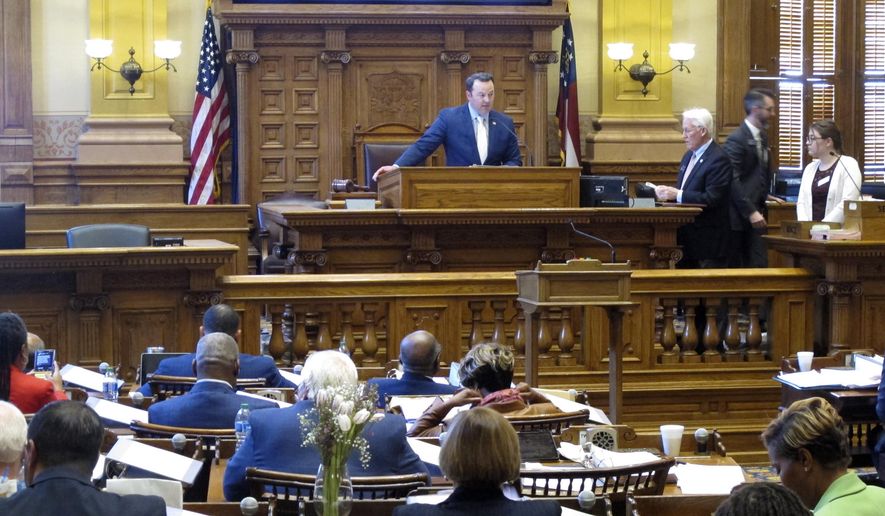The image depicts a detailed scene from the United States Senate. Central to the scene is a man standing at a large, ornate wooden podium, dressed in a blue suit jacket, light blue shirt, and white tie. The man has short hair and is addressing the assembly. Behind him is a grand wooden backdrop adorned with intricate carvings, flanked by two lit lamps on either side. 

To the right of the podium stands an older gentleman, distinguished by his white hair and dark suit, likely wearing glasses. He is holding an object in his hands and appears to be paying close attention to the speaker. There is movement in the background with other individuals walking around; one notable figure includes a woman in a white top who is also focused on the central speaker.

In front of the podium is an ornate wooden guard railing and a smaller podium intended for another speaker. The audience consists of people seated in wooden chairs, all facing the man at the central podium. A notable detail includes a clear glass vase with white flowers and baby's breath, positioned slightly to the left on a table. The flowers, including white tulips with green stems, add a delicate touch to the otherwise formal setting. Additionally, a silver microphone peeks out from the right side of the image, highlighting the formal nature of the proceedings.